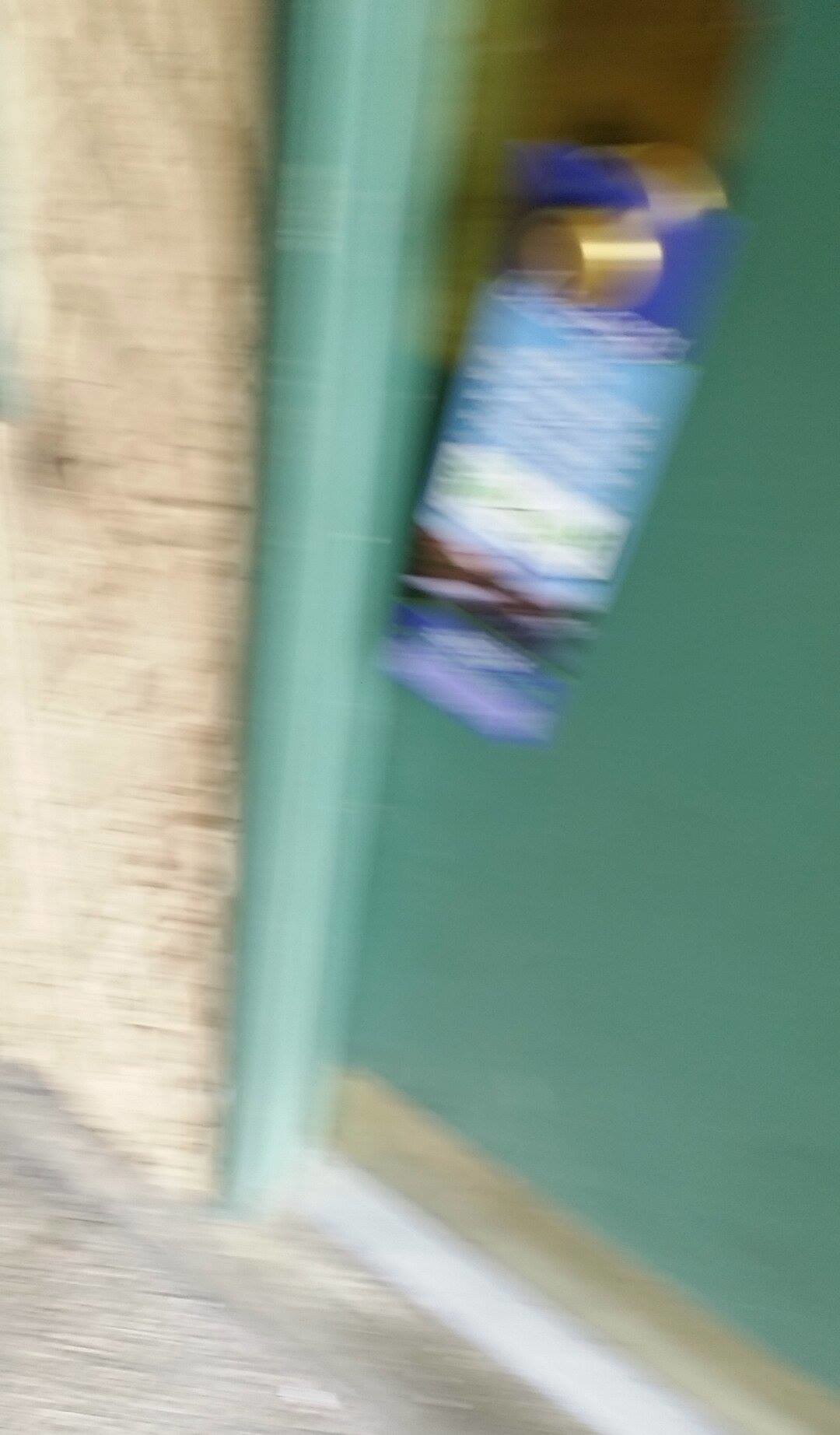The blurry image depicts a sage green door with a gold doorknob and a blue pamphlet attached to the handle. The surrounding wall is composed of textured beige concrete, suggesting a motel setting. The door features a gray strip at the bottom, followed by a white segment beneath that. Though the overall image lacks clarity, the concrete ground appears streaked due to light reflections, adding to the blurry effect. The blue pamphlet hanging on the doorknob contains white and green text and an image resembling mountains, but the blur makes the details unreadable. The building’s exterior is characterized by a textured, multi-colored wall, enhancing its dimensional appearance.